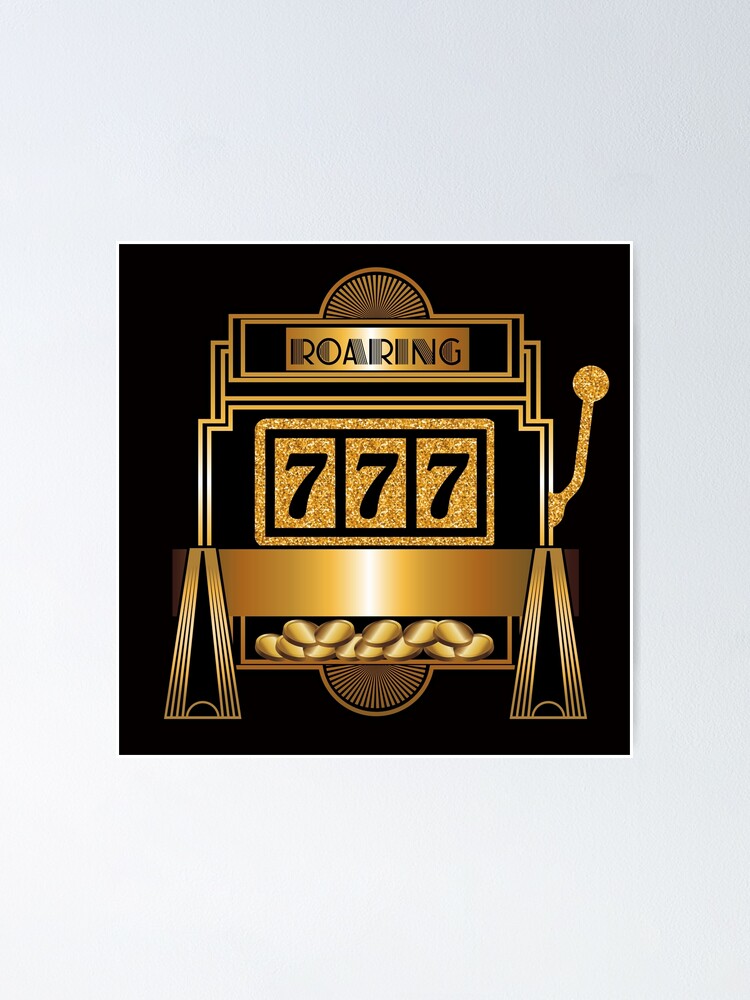The image depicts a minimalistic Art Deco-style slot machine entirely in gold against a black background. At the very top, there is a raised half-circle, resembling a fan symbol typical of such machines. Directly beneath that, the word "ROARING" is prominently displayed in black text on a gold rectangular background, encased in gold trimming. The slot machine features three metallic, shiny gold slots, each displaying a gold-inlaid '777', indicating a jackpot win. Below the slots, there is another gold rectangle with a white, shiny light, signifying the jackpot. Beneath this is an overflowing payout tray filled with coins. A similar raised half-circle motif is present at the bottom of the machine. To the right, there is a lever in the same gold, metallic style, completing the layout. The entire machine stands out vividly against the black background, embodying a sleek, luxurious aesthetic.